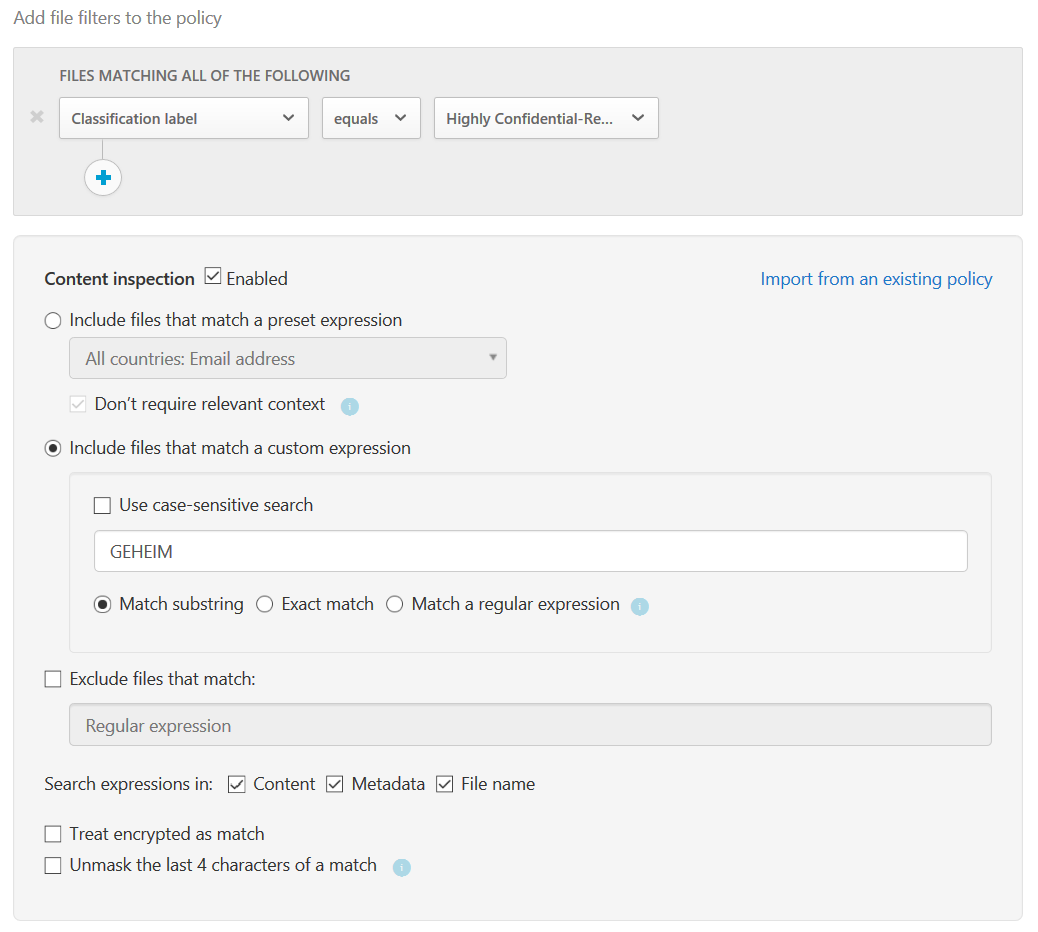**Caption:**

On a light gray background, the top of the interface shows the text "Add File Filter to the Policy." Within this gray box, there is the heading "File matching all of the following" with an "X" icon below it. Underneath, a drop-down menu is displayed, labeled "Classification Label," accompanied by a white circle containing a blue plus sign. Next to this, a smaller drop-down menu reads "Equals," followed by a larger drop-down menu indicating the option "Highly Confidential."

The section below is titled "Content Inspection," featuring a checkbox labeled "Enabled." Adjacent to this, a blue hyperlink states "Import from Existing Policy." Further down, text reads "Include files that match a preset expression," followed by a drop-down menu labeled "All countries email address" with a checked box beside it. The next line reads "Don't require relevant contacts," and below it, a checked circle accompanied by the text "Include files that match a custom expression."

The final section within this box displays an unchecked box labeled "Use case sensitive search," with a text box below it containing the text "GFHHM."